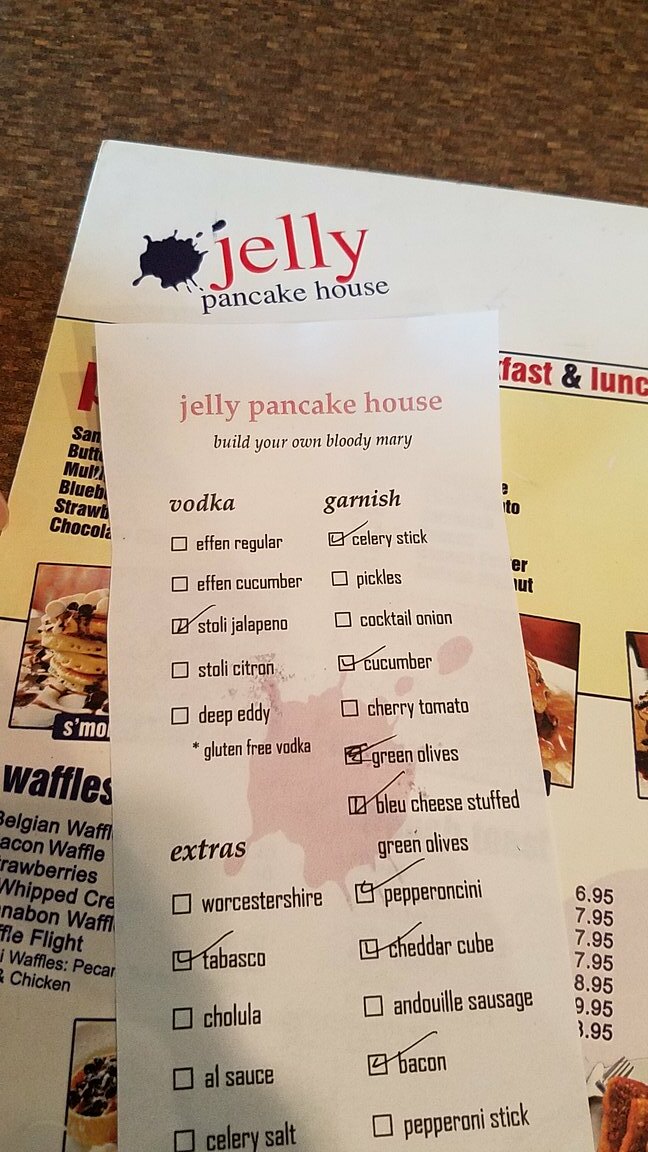This image showcases a table at Jelly, a popular pancake house, featuring a detailed view of the menu and a customized order. Dominating the background is a vibrant menu that highlights the restaurant's breakfast and lunch offerings, with an emphasis on their specialty waffles. 

Above the menu, there's a distinctive "Build Your Own Bloody Mary" checklist that allows patrons to personalize their drink with a variety of ingredients. The checklist includes an extensive selection of vodkas, along with a diverse array of garnishes such as celery sticks, pickles, cocktail onions, cucumbers, cherry tomatoes, green olives, blue cheese, pepperoni, cheddar cubes, sausages, bacon, and pepperoni sticks. Additionally, patrons can enhance their Bloody Mary with extras like Worcestershire sauce, tabasco, cheddar, and celery salt, some of which have already been selected on the docket.

The scene is a testament to Jelly's attention to customization and variety, offering a unique and tailored dining experience.